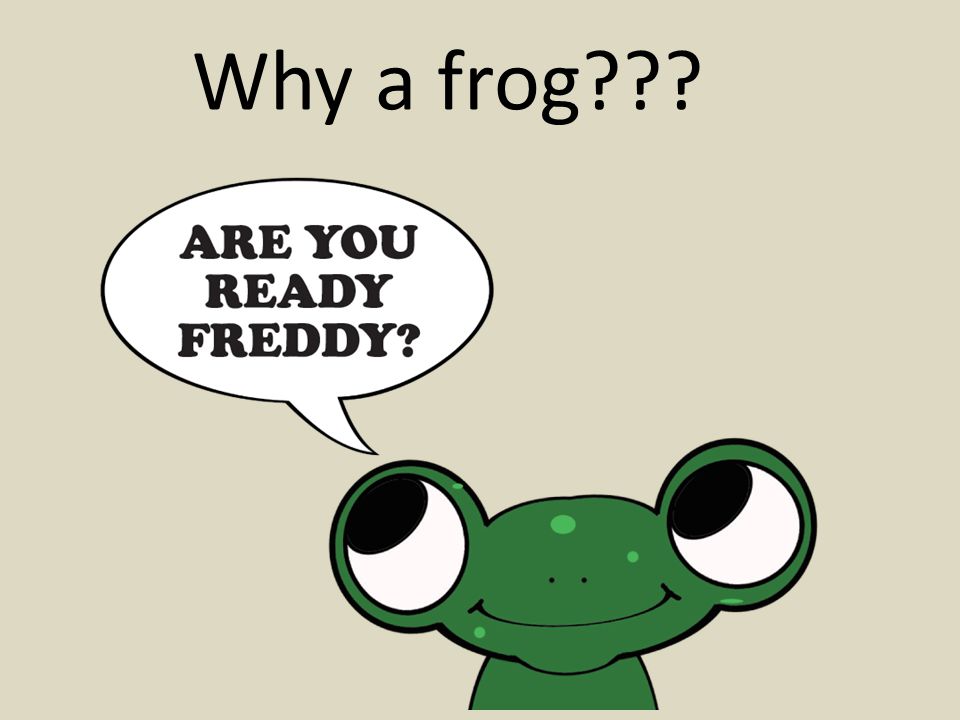The image features a rectangular poster suited for a child's room or classroom, set against a light cream or tan background. At the center of the image is a green animated frog, depicted from the shoulders up. The frog has a cheerful expression, with oversized, circular eyes placed on either side of its oval-shaped head. The pupils of its eyes are looking upwards and to the left. Small black points represent its nose, and light green speckles are dotted across its face and neck. Emerging from the frog's eyes is a thinking cloud that contains the text "Are you ready Freddy?" in bold black print. Above this, at the very top of the image, is prominent text reading "Why a frog???" in black print.